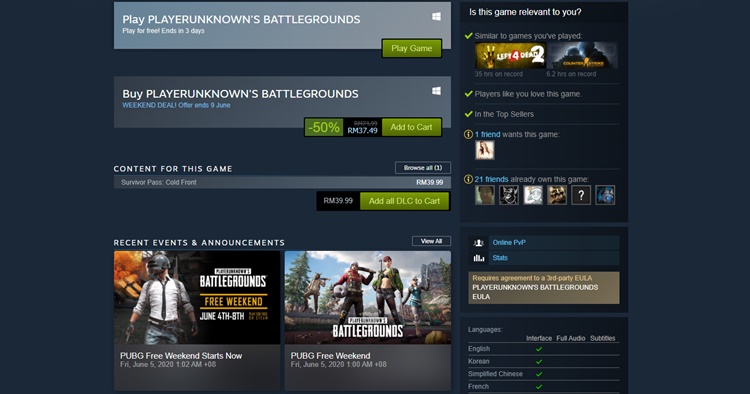This image is a detailed screenshot of a desktop displaying the Steam application, specifically the store page for the game "PlayerUnknown's Battlegrounds." The desktop screen is wide and tall with a solid background. At the top, partially to the left, there is a gray banner that houses the Windows icon, indicating the platform compatibility. Within this banner, there's a small, somewhat hard-to-read notification about something ending in three days. 

Below this, there's a noticeable green "Play Game" button on the lower right of the banner. Immediately under this banner, there's another lighter gray section highlighting a 50% discount offer, with "50% off" and "add to cart" options both marked in green. Further down, another gray banner provides an option to "Add all DLC to cart" in a green button.

Beneath these sections, the screenshot shows two promotional images advertising different aspects of the game, such as a "Free Weekend" event. On the left side of the screen, there is a column dedicated to similar games, making comparisons to titles like "Left 4 Dead 2." This section also displays the number of friends who own the game, current trends, and additional game statistics.